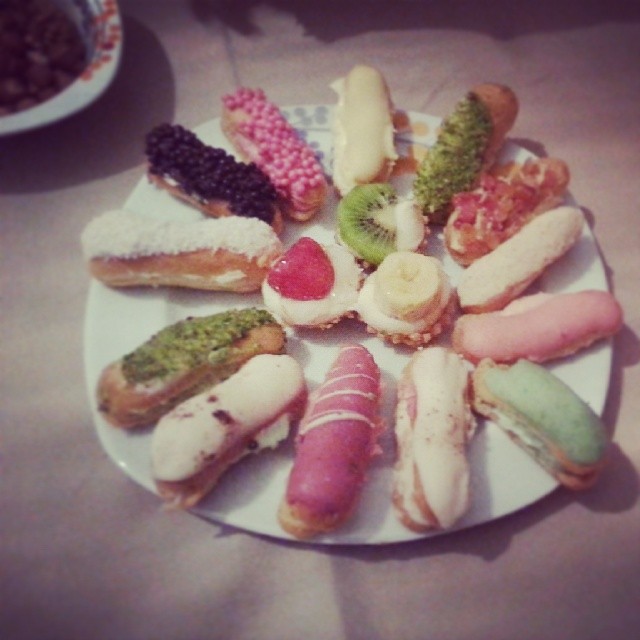The image showcases a white, slightly misshapen round plate, set on a white linen tablecloth, viewed from a top-down angle. Arranged in a circle around the edge of the plate are various oblong pastries, each uniquely decorated. Starting from the top middle and moving clockwise, there's a plain white pastry, followed by one with pistachio frosting. Next is a pastry adorned with chunky pink-orange candy on top of a thick creamy sauce. Then a pink-topped pastry, followed by another pistachio-frosted one. Continuing around, there's a white pastry with brown speckles, a hot pink pastry with white stripes, a white one with dark red drops, and one with dark black orbs. Additionally, there's one with hot pink orbs and another finishes the circle with what appears to be coconut frosting.

In the center of the plate are three smaller, round pastries, each with a distinct topping: the left one features a strawberry slice, the top middle one has a slice of kiwi, and the bottom right one is topped with a banana slice. Some pastries also have cream bases with different fruits and frosting, adding to the variety and visual appeal. Notably, someone has taken a bite out of one of the green-frosted eclairs. Overall, the image captures an enticing assortment of beautifully decorated desserts.